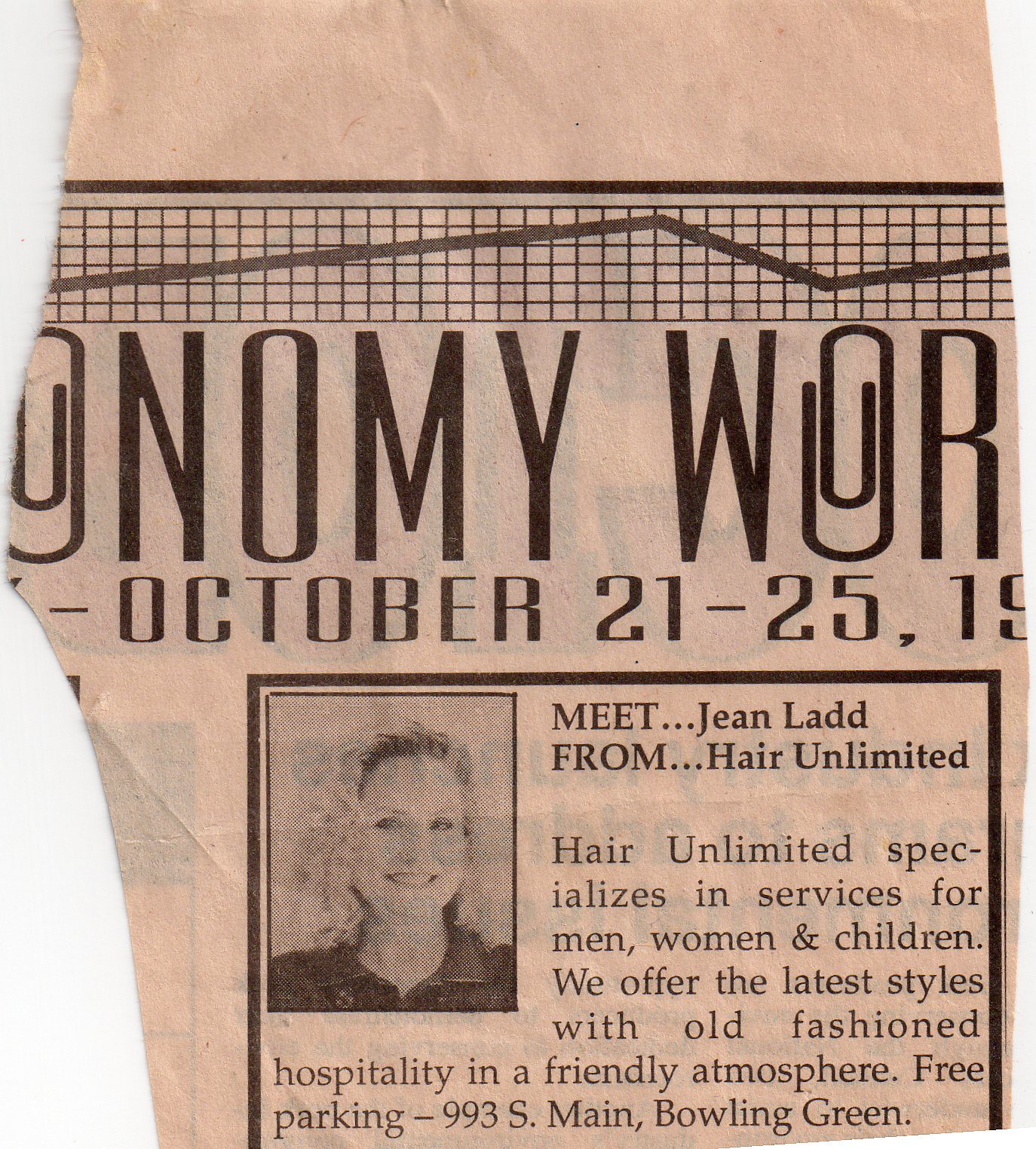This image depicts a weathered and slightly browned black-and-white newspaper clipping, featuring a jagged, ripped corner on the left side. At the top, there is a partial headline with the visible letters "N-O-M-Y" and "W-O-R," which likely spelled out "Economy World." Below the headline, the dates "October 21-25" are partially visible. Near the upper part of the clipping, there is a decorative border resembling a graph, running from the lower left, rising to the upper center, descending to the lower right, then rising again. Underneath the dates, a box contains a picture of a smiling blonde woman with curly hair parted to the side, wearing a polo shirt. The accompanying text reads: "Meet Jean Ladd from Hair Unlimited. Hair Unlimited specializes in service for men, women, and children. We offer the latest styles with old-fashioned hospitality in a friendly atmosphere. Free parking, 993 South Main, Bowling Green."